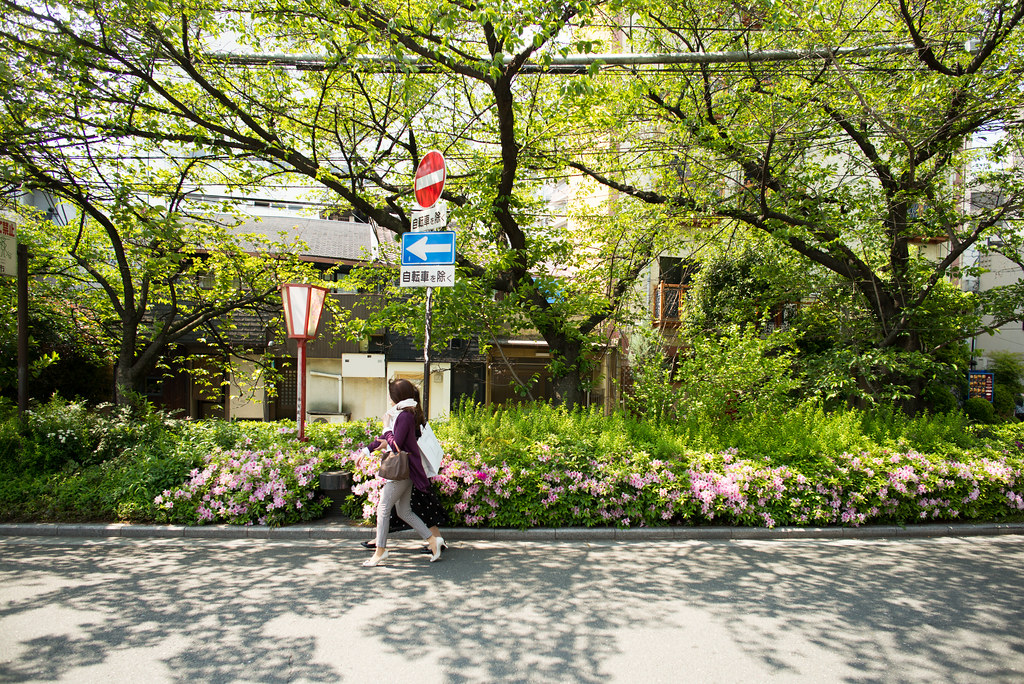In the image, two women are walking side by side down a shady street, flanked by lush greenery and urban elements. The woman on the left is dressed in white high-heeled shoes, gray slacks, a white turtleneck, and a purple jacket. She also carries a white bag over her back. The woman next to her, whose full attire isn't completely visible in the image, wears black flat shoes. The street appears to be gray concrete with shadows from tall trees that almost obscure the sun, some of which have grown into the electrical wires overhead.

To their right, there's a vibrant garden area with abundant pink and white flowers among the bushes and several large, wind-swept trees. They are passing by a street sign with a big blue arrow pointing to the left, topped by a red stop sign, both written in what seems to be an Asian language, possibly Korean or Chinese. A large white concrete building, possibly residential, and several houses that appear older and slightly dilapidated form the backdrop. This rich urban landscape, likely in China, provides a picturesque setting for their walk.